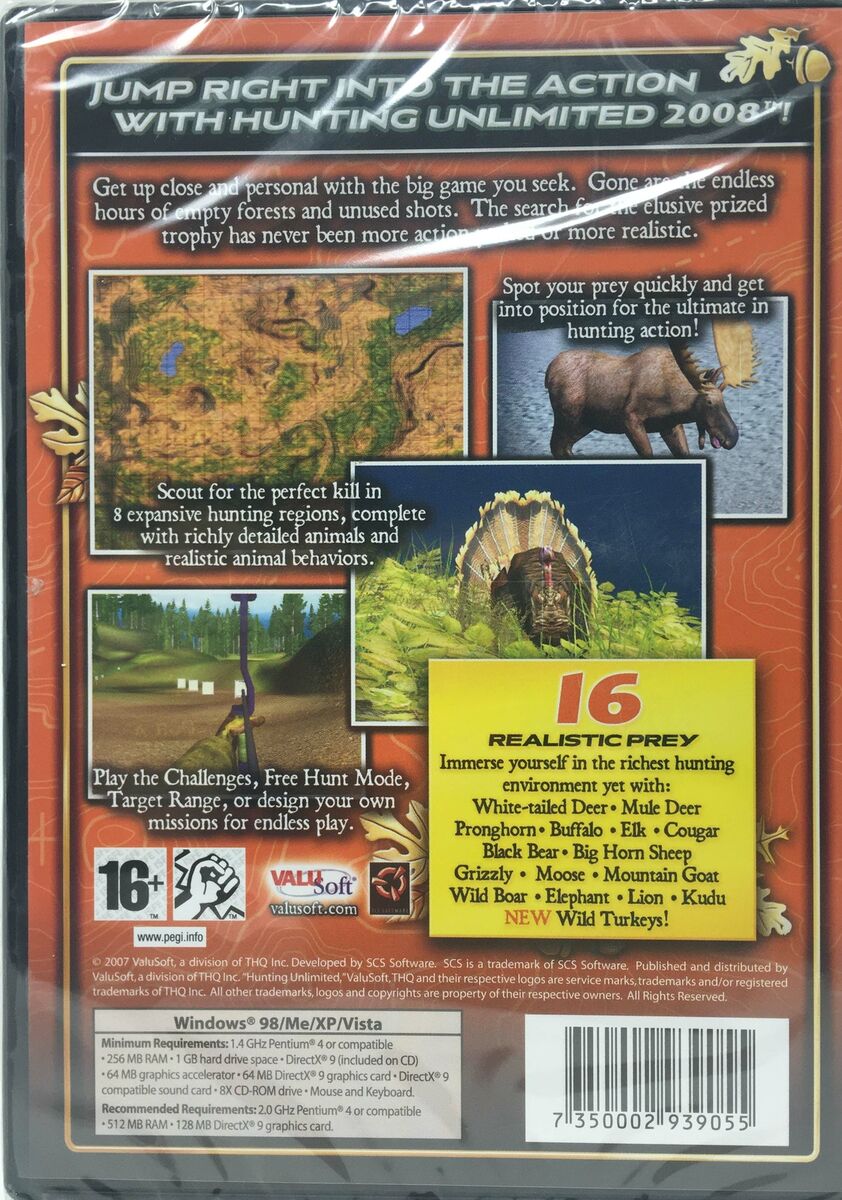This is a detailed color photograph of the back packaging of the computer game "Hunting Unlimited 2008." The package prominently features a red and black design and targets a mature audience of 16 years and older. It showcases an exciting tagline at the top, "Jump right into the action with Hunting Unlimited 2008." The image highlights the key features of the game, including 16 realistic prey such as white-tailed deer, mule deer, pronghorn, buffalo, elk, cougar, black bear, bighorn sheep, grizzly, moose, mountain goat, wild boar, elephant, lion, kudu, and new wild turkeys. The game also allows for various hunting weapons, including guns and a crossbow. The back cover of the package includes three square images: a map, a moose, and what appears to be a dinosaur. Detailed technical specifications, including Windows 98 requirements, are listed alongside a barcode at the bottom.